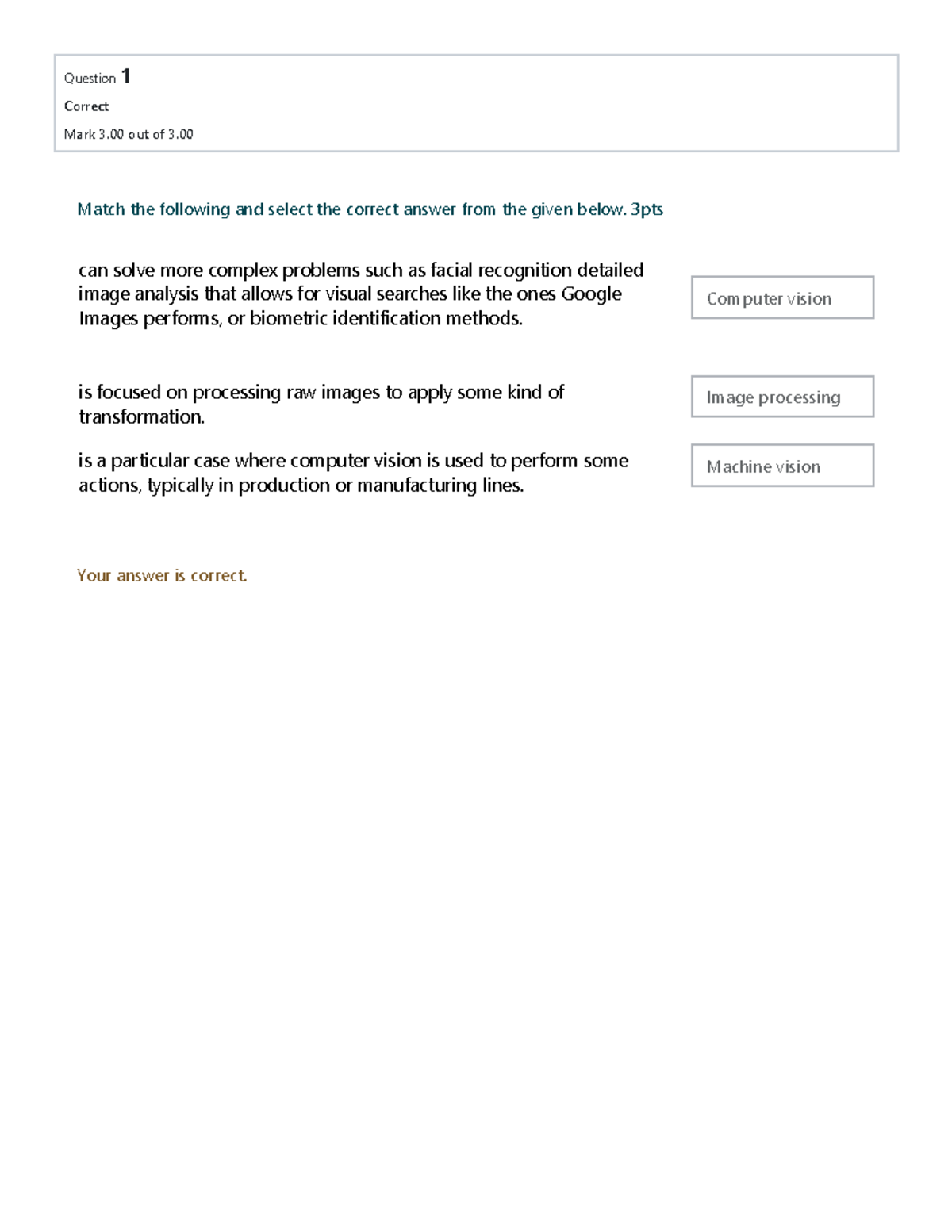An image displays the results of a completed question from a digital test. The interface presents "Question 1" at the top, indicating it was correctly answered with a score of three out of three. The question tasked users to match statements with the correct terms: "computer vision," "image processing," and "machine vision." 

The three statements describe:
1. The ability to solve complex problems such as facial recognition, detailed image analysis, and visual searches similar to Google Image or biometric identification.
2. The processing of raw images to apply some kind of transformation.
3. Using computer vision to perform specific actions, typically in production or manufacturing lines.

The answers provided are:
- Computer Vision
- Image Processing
- Machine Vision

These answers are visually presented in blue text encased in small gray boxes, while the question text is in black. "Match the following" is highlighted in blue as well. At the bottom of the screen, there’s a message in a brownish-gold font confirming the correctness of the answer, stating, "Your answer is correct." The system presumably tracks the progress of the user as they navigate through the test.